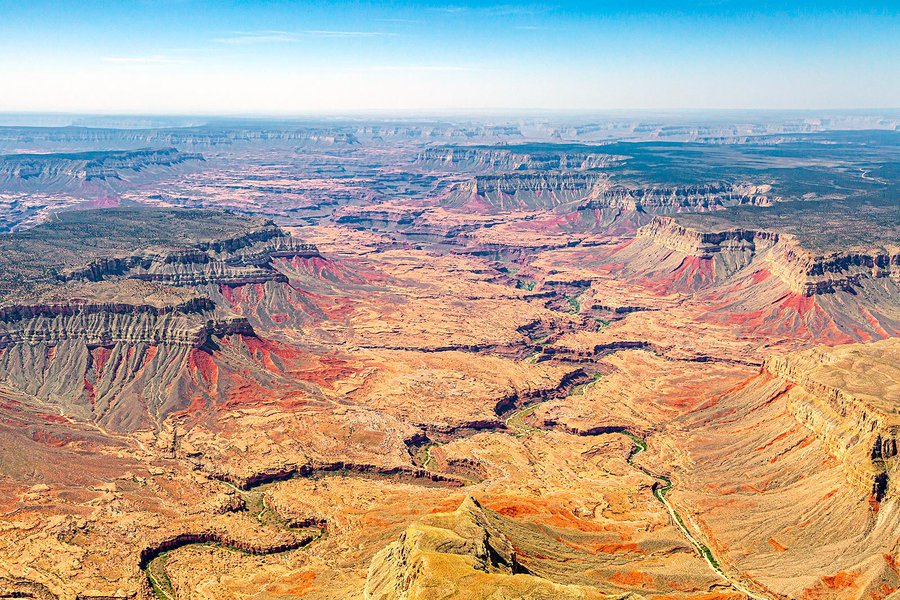This detailed aerial image captures a vast, sweeping canyon landscape, resembling the Grand Canyon or a similar formation in Utah or Nevada. The terrain is marked by steep cliffs and mesas, showcasing distinct geologic layers. The predominantly light brown ground is interspersed with hints of red, yellow, and orange, creating a vibrant desert palette. Amidst this barren expanse, one can trace the ancient, winding patterns of dried riverbeds snaking through the canyons. These dried-up rivers branch off into smaller channels, leading into a larger cavernous area that appears cracked and weathered. Sparse patches of grass persist on the elevated platforms. The distant horizon is hazy with a blend of blue and white, enhancing the infinite reach of this majestic landscape.